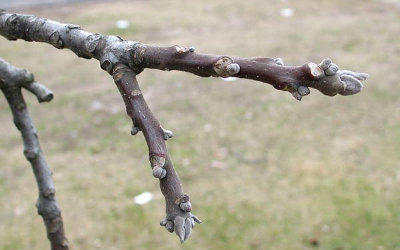This close-up photograph captures a tree branch devoid of leaves, extending from the left side of the frame towards the right. The main branch bifurcates into two smaller sections, both of which exhibit a lighter, purplish hue contrasting the gray, more mature branch they originate from. These smaller branches are tipped with budding formations, hinting at the emergence of new growth, possibly flowers or leaves, indicative of springtime. The branch itself features light gray nodules, adding texture to its mostly brown and gray appearance. The background, heavily blurred to emphasize the branch, reveals patches of dried and green grass, with no text or labels to distract from the natural elements captured in the photograph.